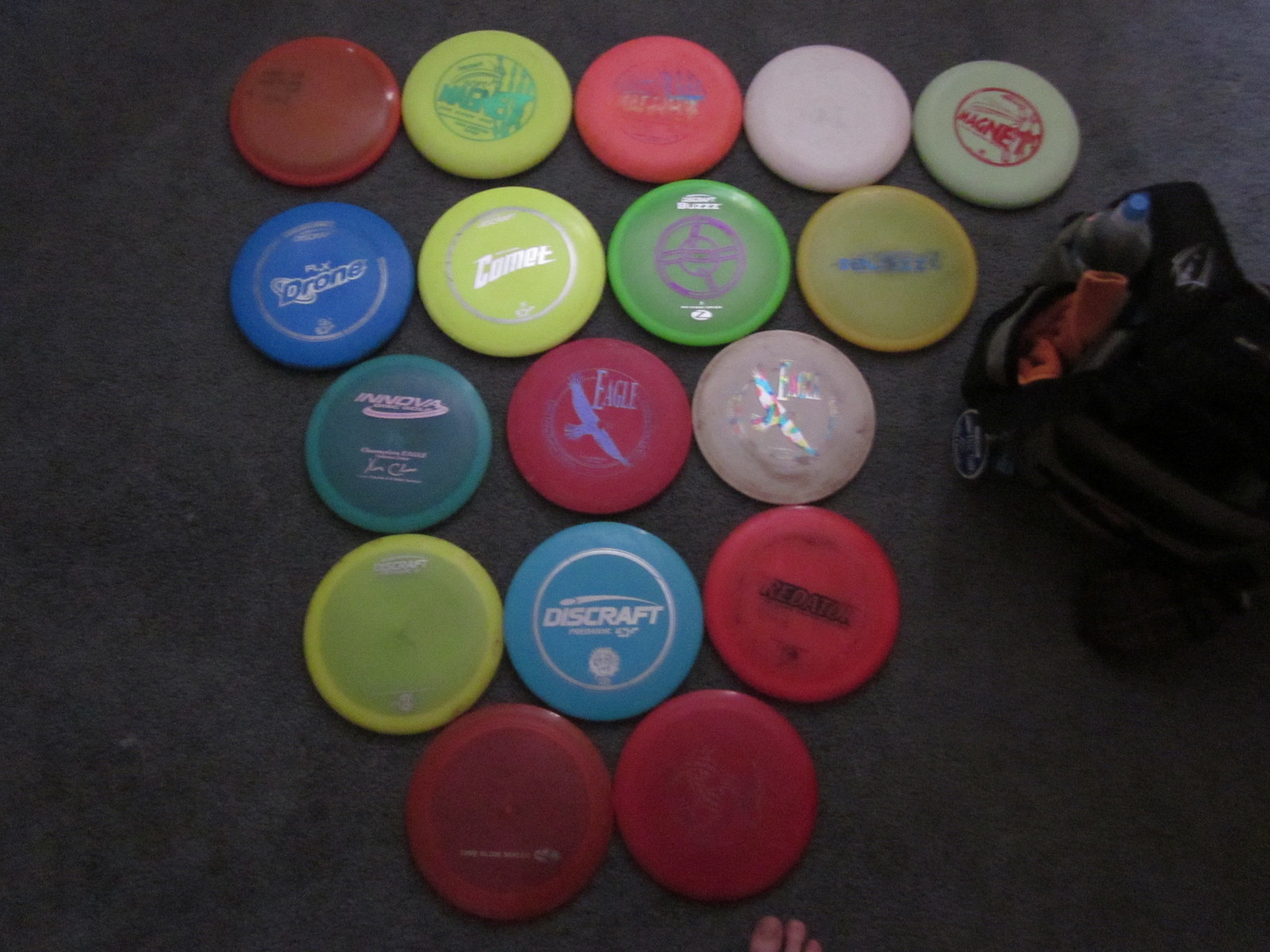The image displays an arrangement of several colorful frisbees on a gray ground, forming a triangular pattern. From bottom to top and left to right, the collection consists of two red frisbees in the bottom row, followed by rows featuring a variety of colors including red, yellow, blue, green, and white. Specific frisbees are marked with brands such as Discraft, Innova, Eagle, Comet, Drone, and Magnet, with notable mentions including a blue Discraft frisbee, a yellow Comet frisbee with silver writing, and a white Magnet frisbee, slightly dirty. A notable detail is the presence of someone's foot at the bottom center of the image, with a visible big toe and two toes. Additionally, a black and white bag containing an orange gear and a water bottle is seen in the top right section of the image.